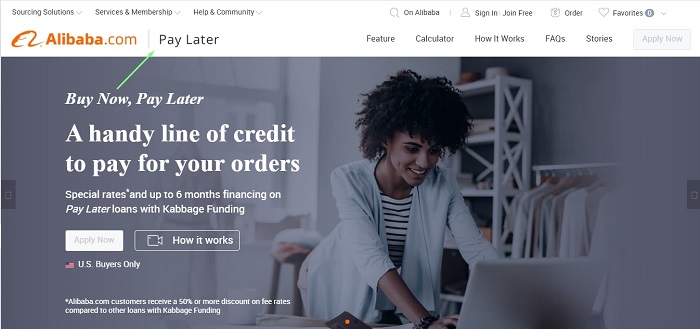**Promotional Webpage for Alibaba.com's "Pay Later" Service**

The promotional webpage for Alibaba.com's "Pay Later" service prominently features a green arrow pointing from "Pay Now" to "Pay Later," highlighting the shift towards deferred payment options. This service offers a convenient line of credit for financing purchases, making it easier for users to manage their expenses.

The navigation menu includes options such as "Solutions," "Services and Membership," and "Help My Community," providing users with various pathways to access financial tools and community support. There are also options to explore Alibaba's financial-free discovery, place orders, handle taxation, and transcribe.

The promotion headline reads "Now Pay Later," emphasizing the flexibility of the service. The central message conveys that users can access a handy line of credit to pay for their orders. Additional details mention special rates and financing options of up to six months on Pay Now loans with CABG funding. 

Two prominent buttons invite user engagement: one labeled "Apply Now" and the other "How It Works." Below these buttons, a disclaimer specifies that the service is available to US buyers only.

Further details at the bottom of the page highlight that Alibaba.com customers receive a discount fee of 50% or more on rates compared to other loans with CABG funding. The background image features a woman smiling and working on a laptop, illustrating the ease of use and satisfaction associated with the service.